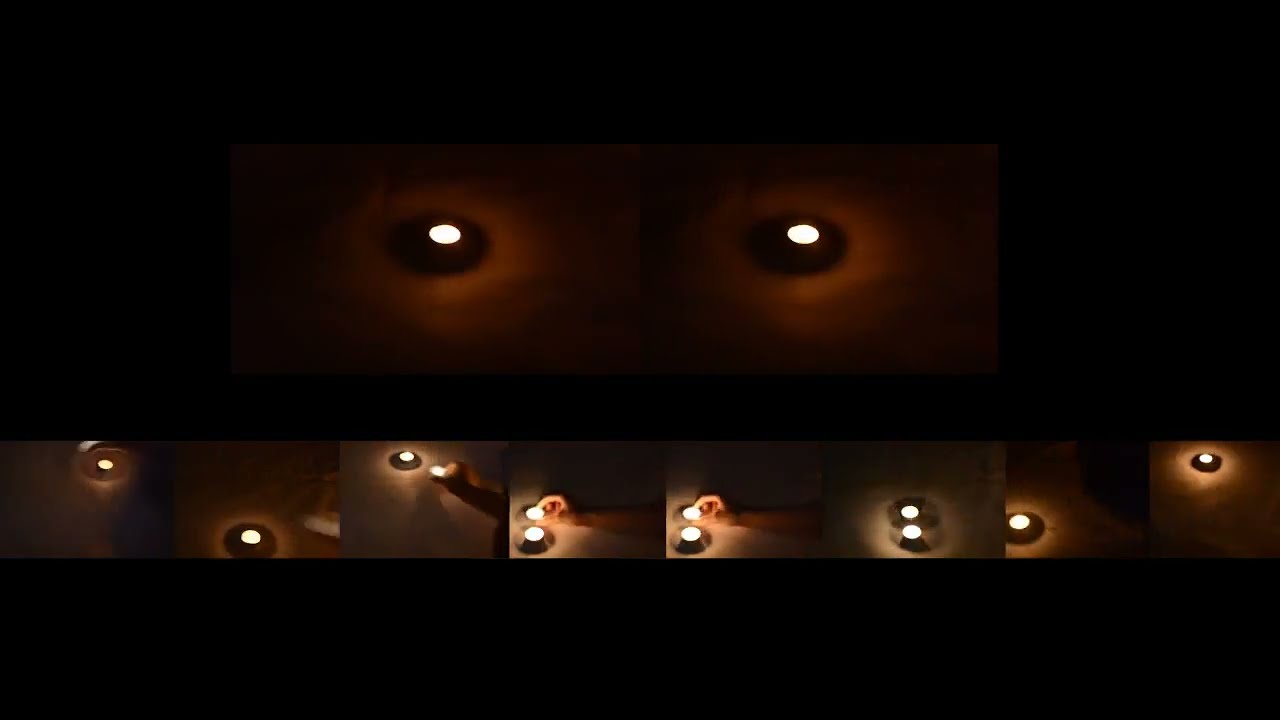The image showcases a series of pictures focusing on lights that resemble eyes. The top portion of the image features two prominent lights situated in the upper right-hand corner, their centers glowing white against a black backdrop, giving the impression of two eyes staring. Beneath these, the image is divided into eight smaller panels, each displaying variations of the light theme. Some panels contain single lights, while others show pairs, with a recurring motif of a hand reaching towards the lights in several instances. The lights are set against a neutral background that transitions from black to a lighter brown. Additionally, a brown table holds a series of tea light candles, some arranged in groups and others standing alone. One panel highlights a book next to the candles on the table. The detailed sequence of lights and hands creates a visual narrative that evokes a sense of interaction with the luminous objects.